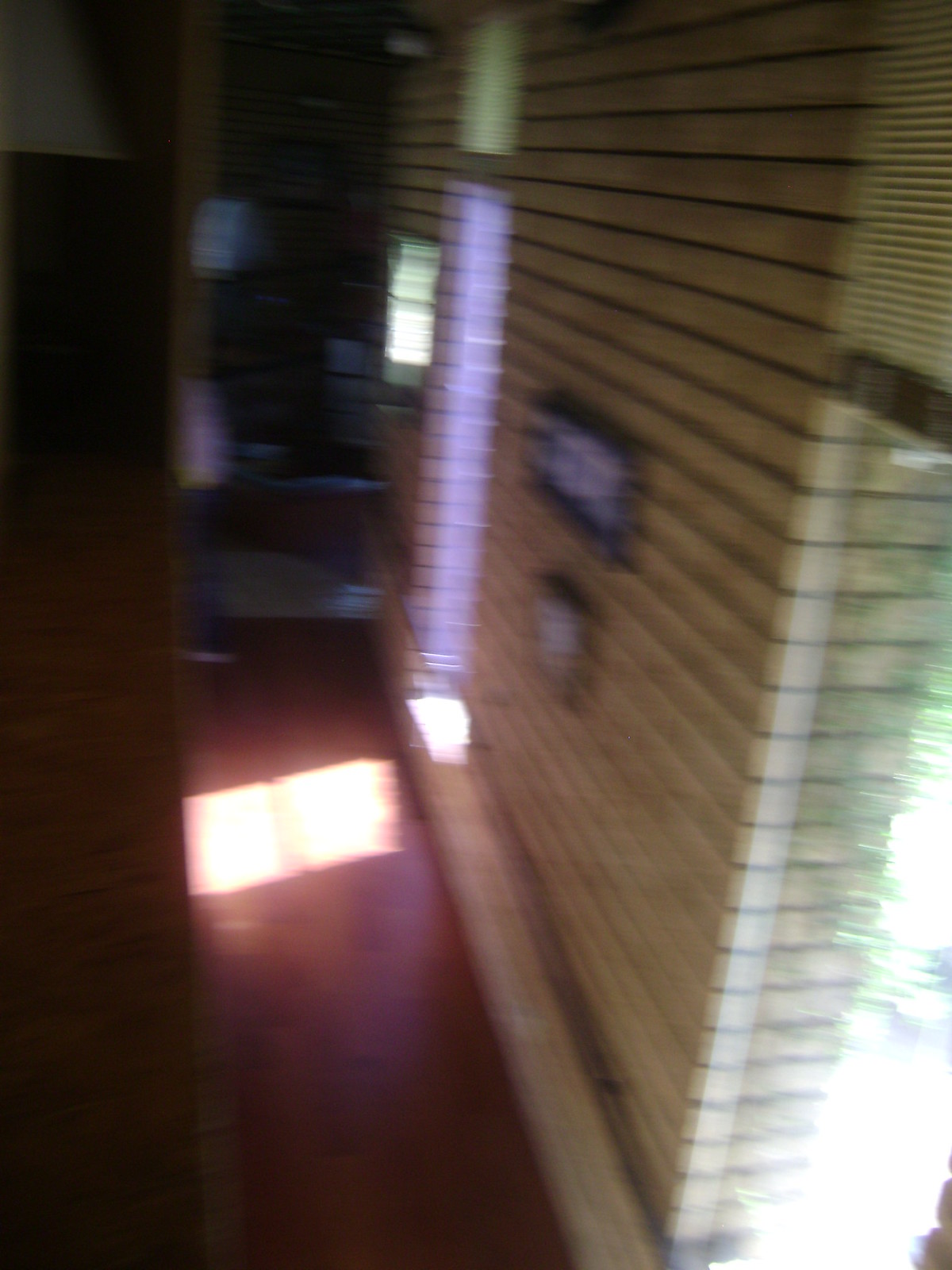An extremely blurry photograph taken in an indoor space, likely a house. The image prominently features a tan brick wall occupying the right side of the frame, adorned with two indistinguishable objects. Flanking the brick wall are two windows with partially raised yellow blinds, approximately three-quarters of the way up. Through the blurry panes, hints of trees are visible outside the right window. A red floor runs centrally up the photograph, leading towards a room in the top left corner, though the blurriness and poor shading obscure further details.